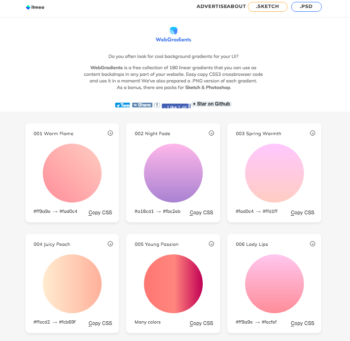This color image, captured from a computer desktop, appears somewhat fuzzy with very small print, making it difficult to read. The image looks to be sourced from a website named "Web Gradients." The layout is square-shaped and features six rectangular sections with white backgrounds, arranged in two rows of three. Each rectangle prominently displays a large circle in the center, each circle filled with a different gradient color. The colors of the circles range from shades of orange to purple, pink, and various transitions in between. Specifically, the gradients include:

1. An orange circle.
2. A purple circle.
3. A pink circle.
4. A light orange circle.
5. A circle with a red hue on the right, fading to orange on the left.
6. A darker pink circle located at the bottom right-hand corner.

In the upper left-hand corner of the image, there is some small text that advertises a website, roughly reading "advertise sketch.sketch.psid".